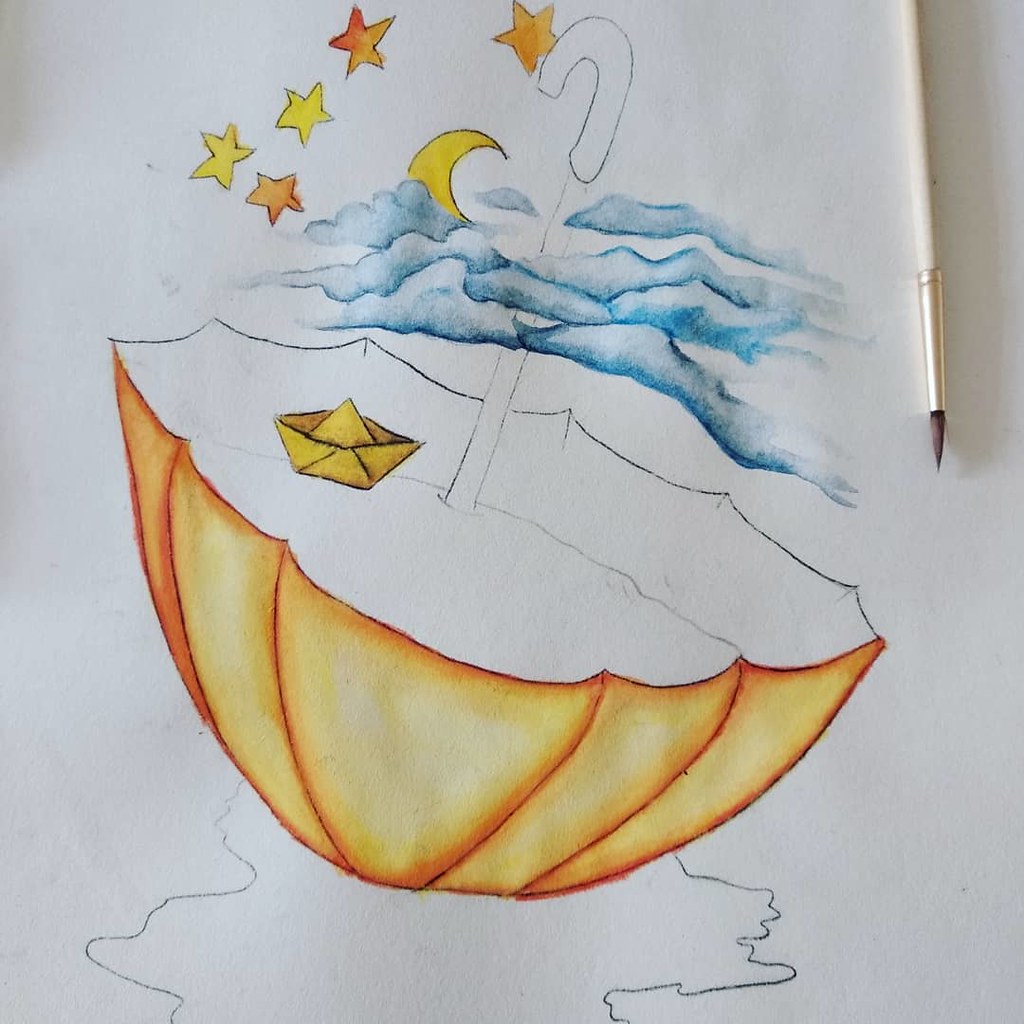### Descriptive Caption:

This enchanting close-up reveals a partially colored painting, likely created on white paper that appears light grayish-lilac due to reproduction. The focal point is an upside-down umbrella, intricately sketched with a fine-tipped instrument. The umbrella, rendered in a soft, light orange hue, deepens towards the edges of its sectioned ribs, while the center remains unpainted. Inside, a possibly uncolored yellow paper boat or hat rests, hinting at an uncompleted interior scene, potentially with water suggested but not yet depicted. 

Above the umbrella, delicate white and blue clouds float serenely in the sky. The handle of the umbrella arches gracefully like an inverted candy cane, ending in a hook. Surrounding this whimsical scene are five stars—three gold and two yellow—accompanied by a charming crescent moon, adding a dreamlike quality to the composition. The overall aesthetic suggests a story suspended in time, a work in progress brimming with imagination and delicate details.